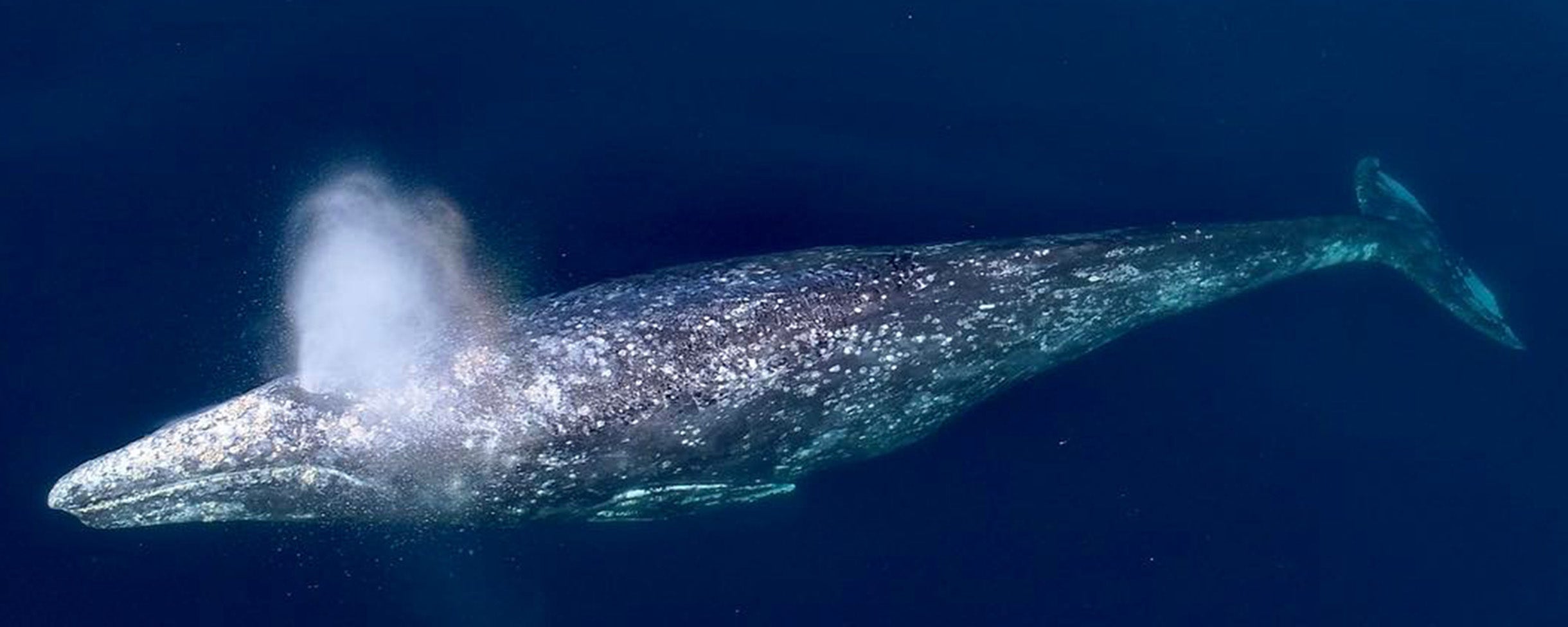In the photo, we see a large, elongated sperm whale submerged in crystal clear, deep blue water. The whale's long, dark gray body is dotted with white spots, suggesting a possible plankton growth on its back. Positioned above its eyes and just before its mouth, the whale’s blowhole is actively spouting water and steam. You can vividly see the spout amidst the dark blue background. The horizontal placement of its tail fins and the flippers located behind its head are clearly visible. The image is likely an overhead shot taken from a boat or a nearby vantage point, capturing the whale's detailed skin texture and body outline as it moves in the deep sea.